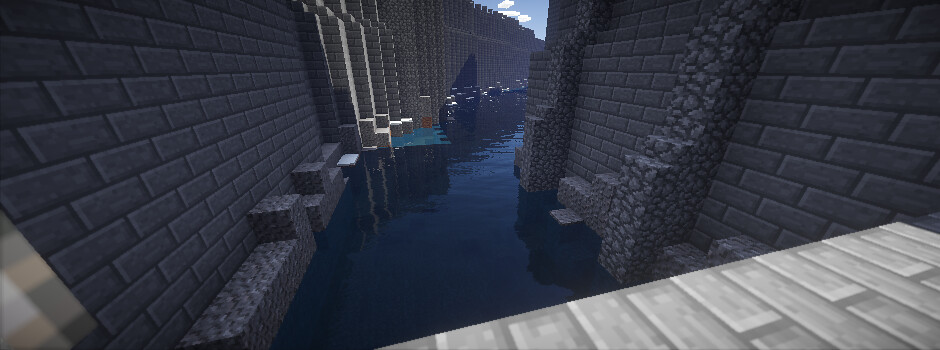This image appears to be a screenshot from a video game resembling Minecraft, characterized by its blocky design. Dominating the scene are structures made entirely of various colored blocks with distinct patterns. In the foreground, there's a light gray block resembling wooden flooring. Adjacent to this, on the bottom left, is an object composed of different shades of brown. Flanking both sides of the image are imposing dark gray stone walls that extend from the front all the way to the back, where they bend around a corner. Above this scene stretches a blue sky dotted with blocky white clouds. The walls enclose a central waterway, which is dark and shiny, less pixelated than the surrounding elements. The middle section of the image features the water, with reflections enhancing its dark blue hue. In the distance, some gold-hued stone structures and a green platform can be seen, adding depth to the intricate virtual landscape.